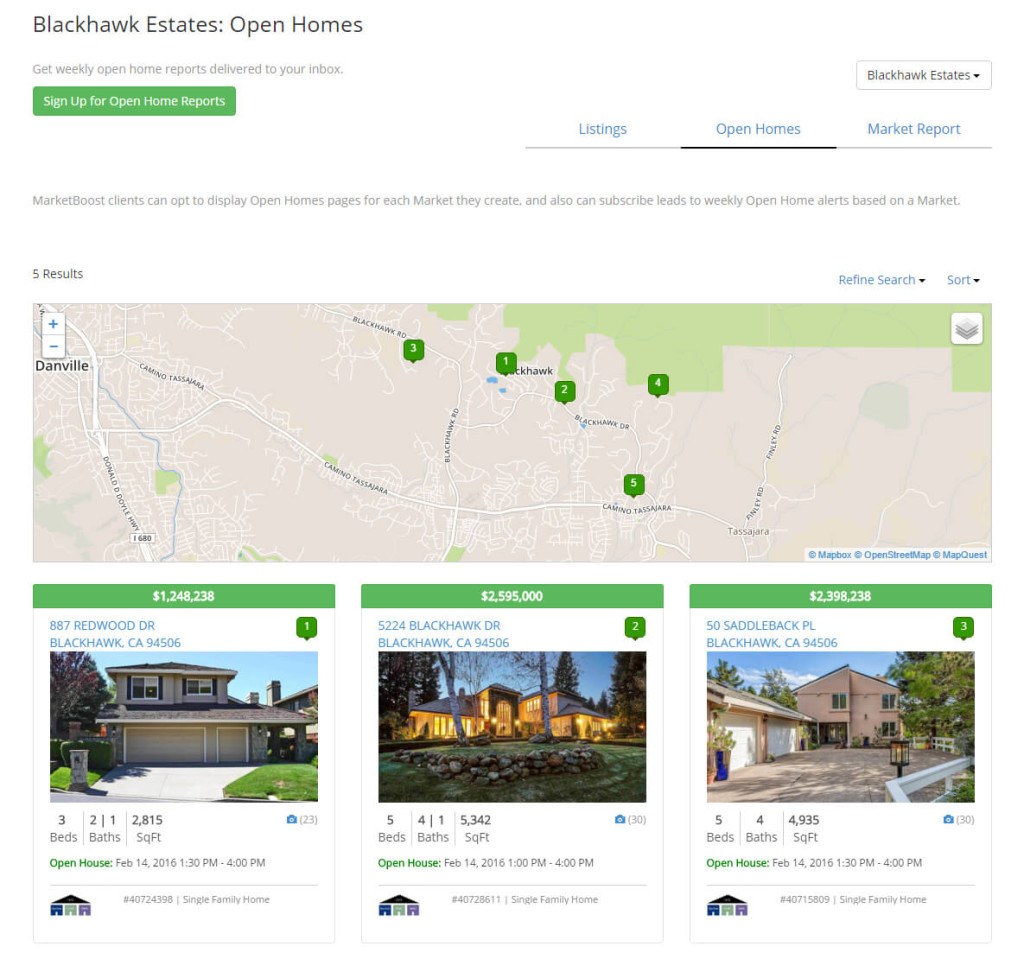A screenshot from a real estate website is displayed, showcasing available properties in Blackhawk Estates. The top left corner features a header in black text reading "Blackhawk Estates: Open Homes," followed by a gray subtext that invites users to "Get weekly open home reports delivered to your inbox." Beneath this text, a green button with white lettering encourages visitors to "Sign Up for Open Home Reports."

On the left side of the screenshot, there is a drop-down menu labeled "Blackhawk Estates" in black text. Below this menu are headers in blue text titled "Listings," "Open Homes," and "Market Report." Further down, a paragraph in gray text explains that "Market Boost clients can opt to display open home pages for each market they create and also can subscribe leads to weekly open home alerts based on the market."

The center of the image features a beige map with white-labeled roads and black text. Numbered points of interest (1 through 5) are visible, while a plus and minus sign for zoom options are located in the upper left corner of the map. In the lower right corner, credits read "Open Box" at "Open Street" "Open MapQuest."

Below the map, three property listings are presented, each in its separate box with accompanying photos and details. To the far left is a property priced at $1,248,238, located at 287 Redwood Drive, Blackhawk, California 94506, featuring three bedrooms and two baths within 218 square feet. The center property is listed at $2,595,000, situated at 2224 Blackhawk Drive, Blackhawk, California 94506, offering five bedrooms and four baths in a 530 square foot area. The property on the right is priced at $2,398,238, found at 50 Center Back Point, Blackhawk, California 94506, and includes five bedrooms and four baths over 493 square feet.